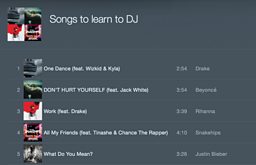A small, blurry screenshot appears to have been captured from either a phone or computer screen. The background is a dark charcoal gray, with white text and small images next to each listed song. The top of the image bears the title "Songs to Learn to DJ," accompanied by a square containing four smaller images that represent some of the songs listed below. 

The songs are numbered from 1 to 5, though the text is difficult to read clearly:
1. The first song is extremely blurred and mostly illegible.
2. "Don't Hurt Yourself" featuring Jack White - possibly by Beyoncé.
3. "Work" featuring Drake - by Rihanna.
4. "All My Friends" featuring an unidentified artist and Chance the Rapper.
5. "What Do You Mean" - by Justin Bieber.

Next to each song title are the track durations and what appear to be artist names. The second song seems to credit Beyoncé, the third references Rihanna, the fourth is too blurry to discern, and the fifth lists Justin Bieber. Despite the poor image quality, the list appears to aim at curating songs for aspiring DJs to learn.